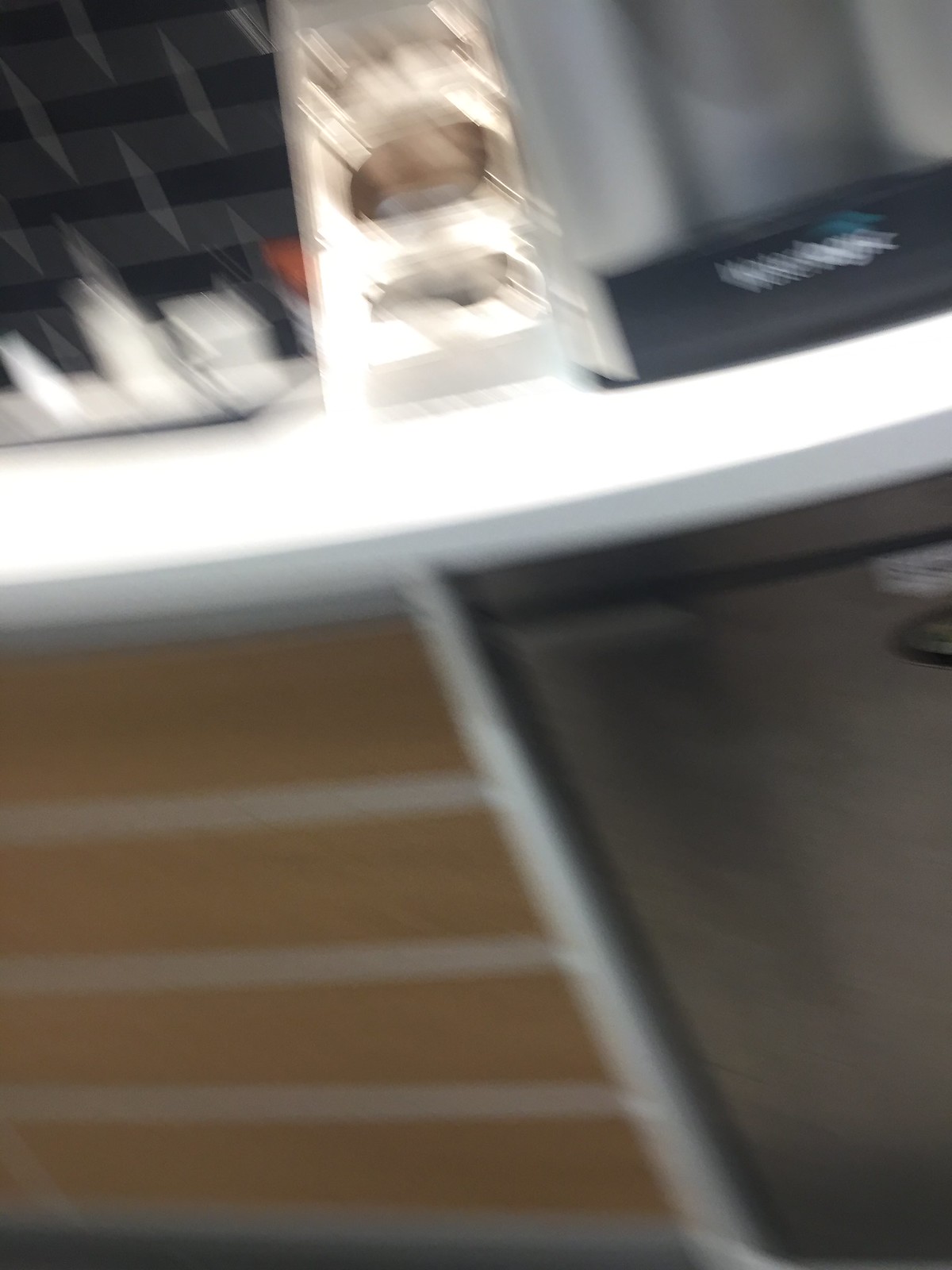This image is a very blurry, grainy photograph depicting what appears to be a break room or kitchen area. The rectangular frame is divided into several distinguishable sections by color and shape, despite the lack of sharpness. Toward the lower left corner, there is a tan area featuring three white horizontal stripes. This tan area seems to be separated by a diagonal line from the lower right section, which is dark gray in color, suggestive of a metallic mini-fridge. Above this area, a white horizontal stripe runs across the image about two-thirds up, resembling a countertop. Positioned on this countertop, there is a rectangular block-like item on the right, possibly a coffee machine like a Keurig. Adjacent to it is a white object resembling a small shelf with openings. To the left on the countertop, there's an unidentifiable white and blurry object, potentially other break room essentials like snacks or plastic cups. The upper left corner is predominantly black with vertical grayish stripes, and the area above the white stripe in the center displays a bright, reflective, ladder-like shape, flanked by black and gray segments with vertical divisions. Despite being indistinct, this setup evokes the image of a common area in an office or hotel.